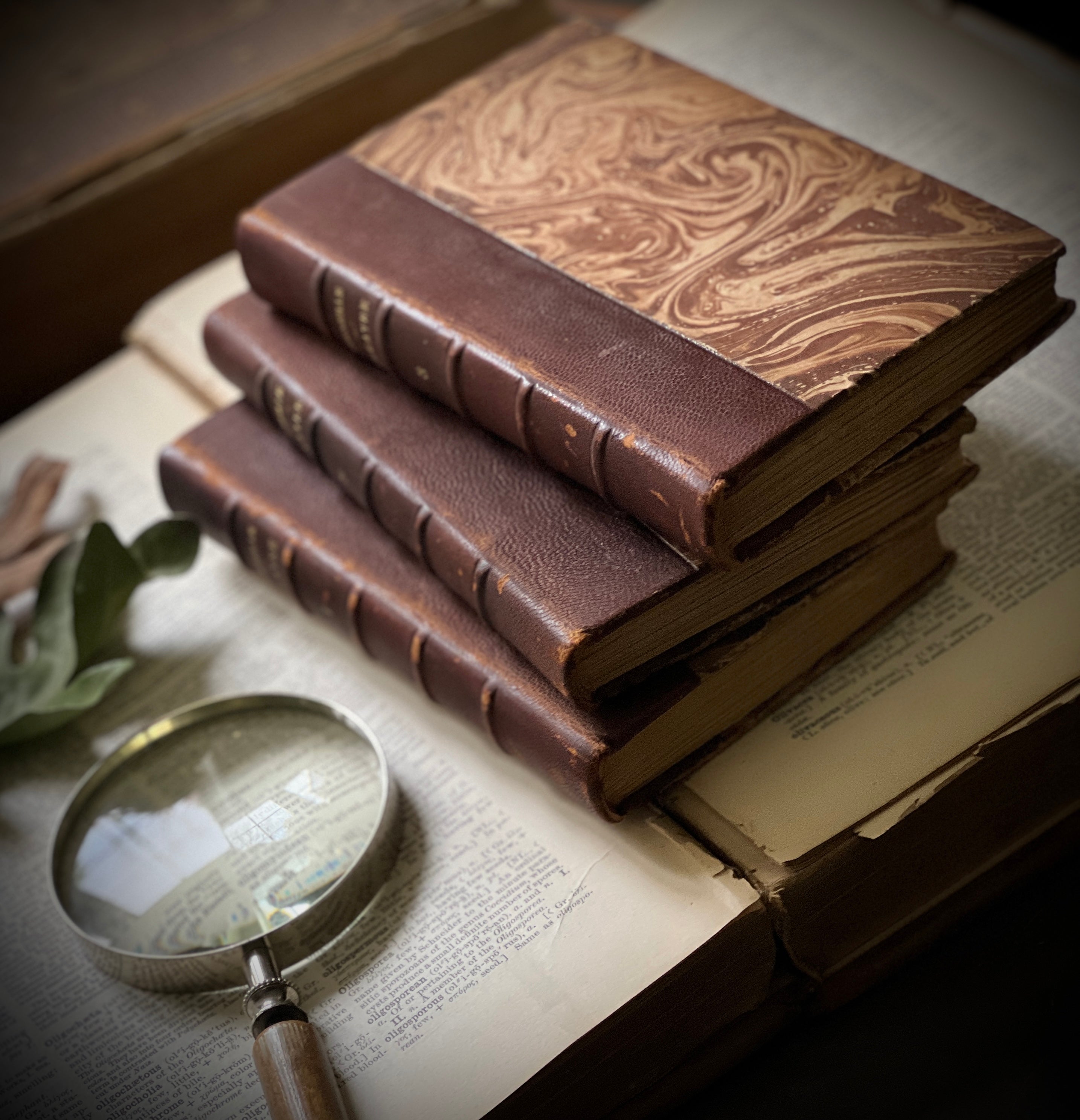This color photograph, ideal for Instagram, captures a vintage, artistic scene from above. At the center, a stack of three leather-bound books with dark red to maroon spines and gold text, slightly out-of-focus and unreadable, are precariously placed atop an open, larger vintage book with black and white text. The covers of these hardbound books feature a classic brown and beige swirly pattern, with one book slightly askew, adding to the picturesque disarray. A silver-rimmed magnifying glass lies over the open pages in the lower left corner, partially covered by a couple of green leaves. The dramatic, soft-focus lighting accentuates the antiquarian charm of the scene, making it a perfect composition for social media. In the upper left, a brown wooden shelf subtly enters the frame, adding depth and context to the tableau.